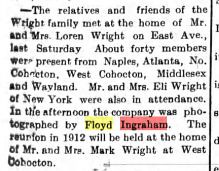The image displays a small snippet from a newspaper article discussing a family reunion of the Wright family. It details that the relatives and friends of the Wright family gathered at the home of Mr. and Mrs. Lauren Wright on East Avenue last Saturday. About 40 members attended, traveling from places like Naples, Atlanta, West Coherenton, Middlesex, and Waveland. Additionally, Mr. and Mrs. Elliott Wright from New York were also present. In the afternoon, the gathering was photographed by Floyd Ingram, with "Floyd" highlighted in yellow and "Ingram" in red. The passage also mentions that the next reunion, planned for 1912, will be hosted at the home of Mr. and Mrs. Mark Wright in West Duponton. A black separating line runs from the top edge to the bottom right corner of the clipping, partially obscuring some text on the right.